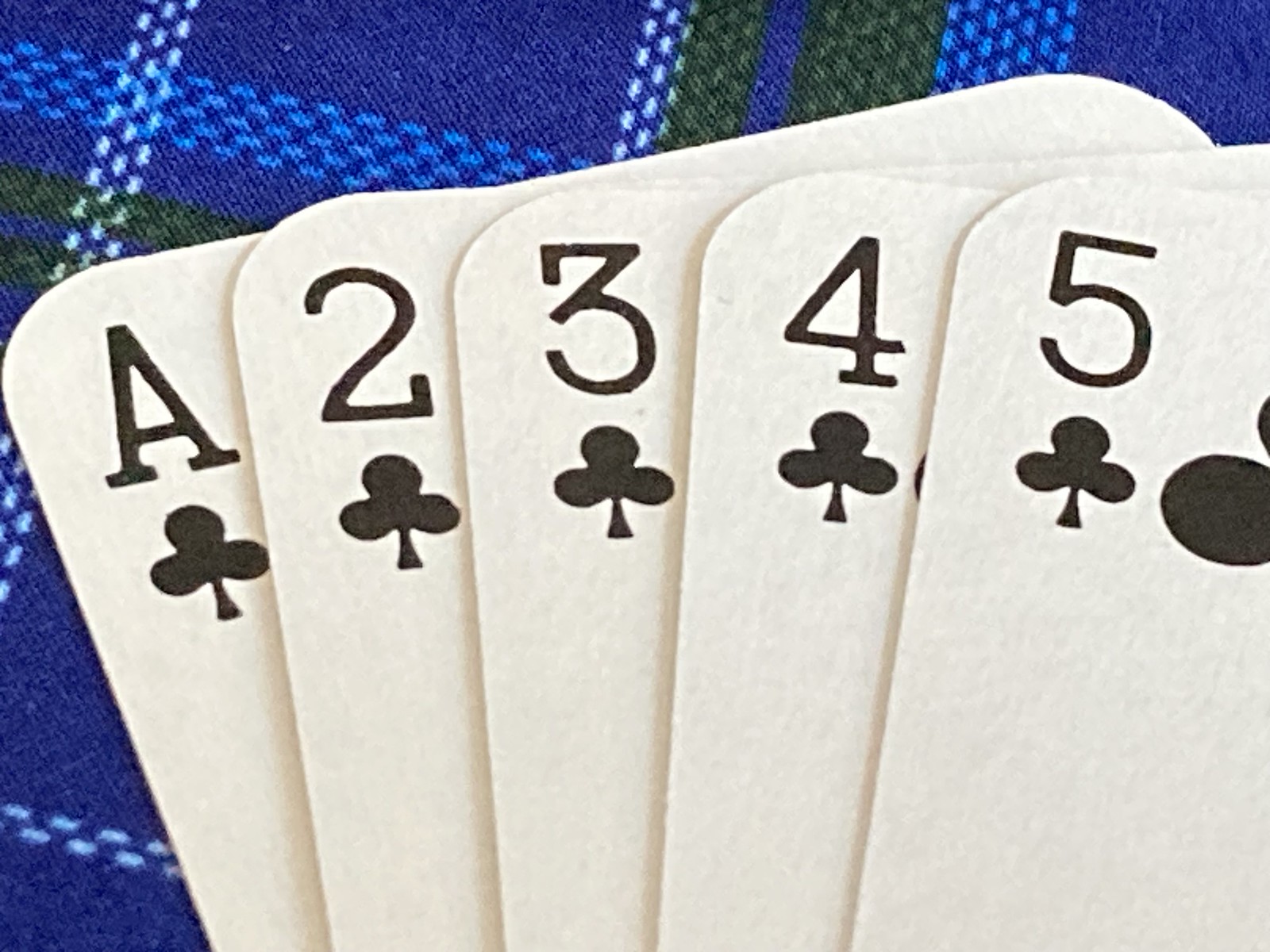This close-up image features five playing cards from a deck, specifically clubs, arranged in numerical order: Ace, 2, 3, 4, and 5. The cards are distinctively round with curved corners, and have a clean white background. Only the top three-quarters of each card is visible, capturing the suit and number positioned in the upper left corner. The cards are set against a blue plaid fabric that contains varying shades of blue, green, and white, suggesting a tablecloth or similar textile. The composition is zoomed in, with the cards occupying the majority of the frame, emphasizing their unique round shape and the intricate pattern of the fabric beneath them.